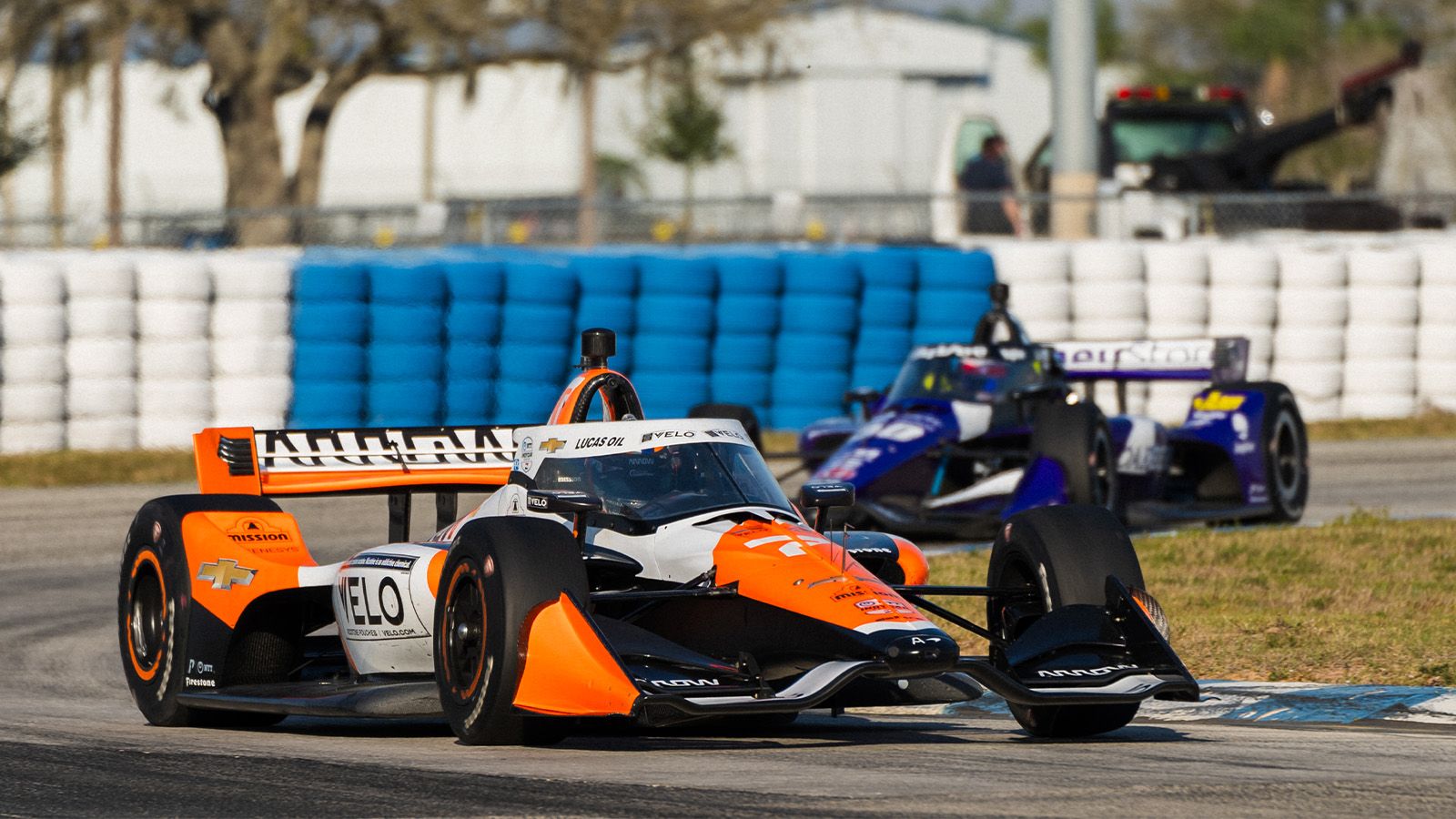This image captures an outdoor racing scene on a rectangular asphalt track featuring two vintage Formula One race cars. The foremost car, an orange and white go-kart with large black tires, is closely followed by a blue and white car of similar design. They are navigating a bend that curves from right to left and back to the right. The race cars are set against a backdrop of blue and white tire barriers, each stack approximately five tires high. Beyond the barriers, the scene includes a grassy strip, white buildings, a tree, a chain-link fence, and the rear end of a tow truck. The vivid colors and combination of elements enhance the dynamic and lively atmosphere of the race track.